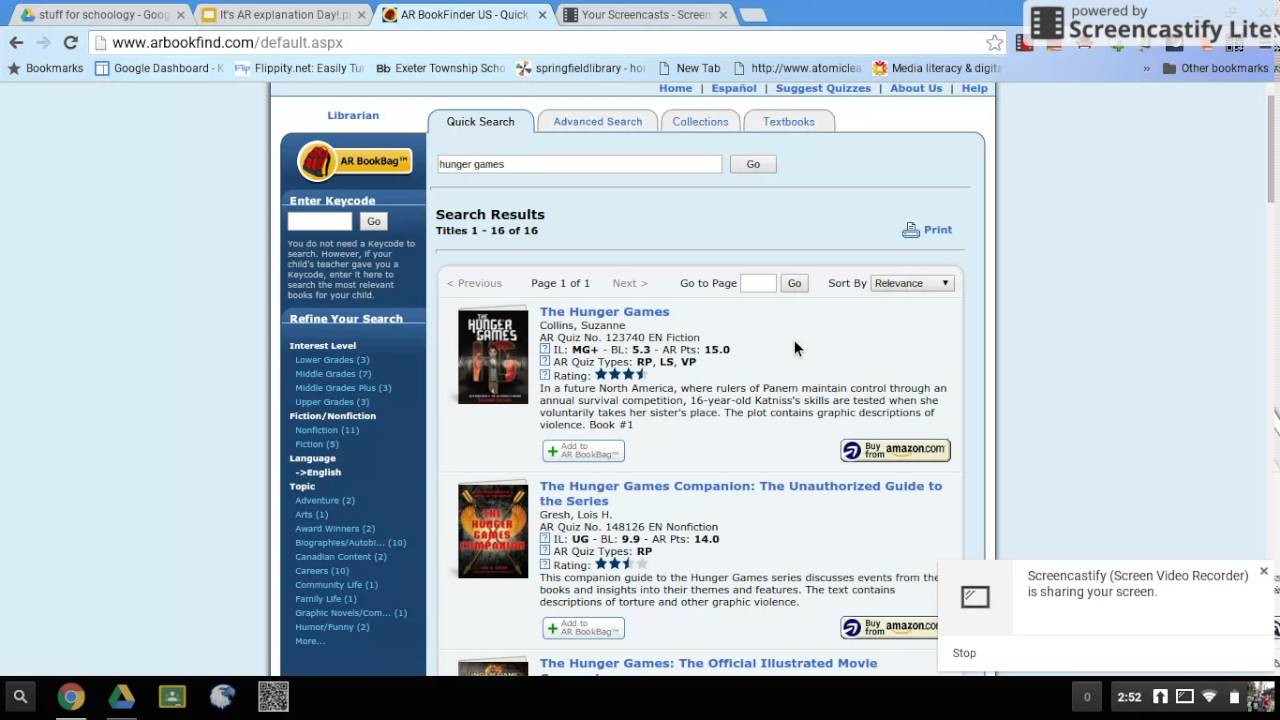### Detailed Caption:

At the top part of the webpage, there are four tabs with the first two appearing in gray, the third one in light blue, and the last one in gray. The first black tab is labeled "School Stuff," followed by the next tab labeled "AR Explanation Day." The third tab, which is light blue, displays "AR Book Finder US," and the final tab reads "Your Screencast." The web browser section is predominantly white, with the URL bar displaying in black text: "www.aofinefine.com/Default.aspx."

Several additional tabs are open within the browser. Listed in black text, these tabs include: "Books," "Google," "Repeated Flippity," "NetXETER Township Springfield Library," "New Tab," "Atomical Media Literacy and Digi," although the text cuts off at this point.

Beneath this, the page features a blue background with a navigation bar at the top. This navigation bar contains links in blue text labeled: "Home," "Suggests Quizzes," "About Us," and "Help." Below this, a white section prominently displays the word "Librarian" in blue.

Following this section, a light blue tab is marked with "Quick Searches" in black text. Other tabs labeled in gray include "Advanced Search," "Collections," "Textbooks," and "Search Results." Within the "Search Results" tab, it lists titles 1 to 16 out of 16.

Highlighted in blue, one of the search results reads "The Hunger Games," with the author listed in black as "Collins, Suzanne." Another result in blue is "The Hunger Games Companion: The Unauthorized Guide to the Series," with the author listed in black as "Gresh, Lois H."